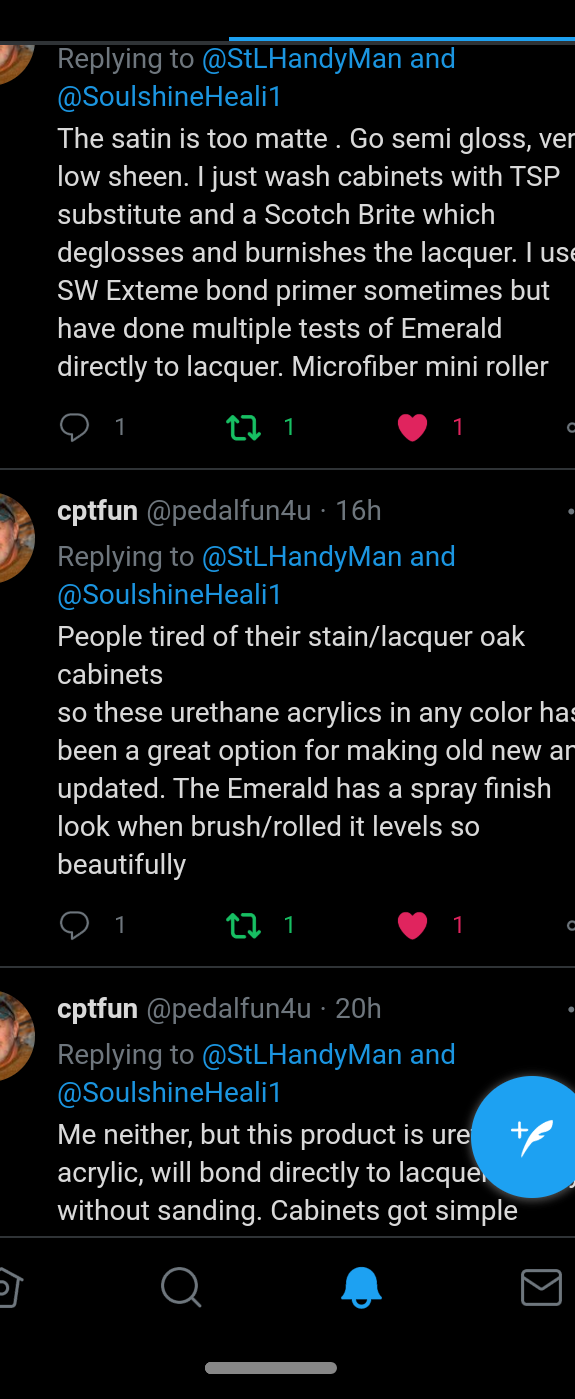Here's a cleaned-up and detailed caption for the image:

---

**Image Description: A Reddit Reply Interface**

The image shows a screenshot of a Reddit post discussion with a black background. The user "Captain Fun" is engaged in a detailed conversation with "Saint Handyman" and "Soulshine Hailing 1" about painting and finishing techniques for oak cabinets. 

1. **Reply from Captain Fun, 16 hours ago:**
    - **Text:** "People try to stain and lacquer oak cabinets. Urethane acrylics, available in any color, have become a popular choice for updating old and new cabinets. The Emerald paint offers a spray finish appearance when brushed or rolled, resulting in a beautiful surface."
    - **Engagement:** 1 comment, 1 share, 1 like.

2. **Reply from Captain Fun, 20 hours ago:**
    - **Text:** "I've used SW Extreme Bond Primer sometimes but prefer testing Emerald directly on lacquered surfaces using a microfiber mini roller. Satin finishes can be too matte or semi-gloss. For prepping, I wash the cabinets with TSP, use Scotch-Brite pads, and avoid burnishing and lacquer buildup."
    - **Engagement:** 1 comment, 1 re-quote (or similar), 1 like.

There is also a semi-cut-off part of the interface, showing a little circle with a quill plus icon, indicating additional options. The home, search, and mail icons at the bottom left of the screen are partially visible, suggesting the interface might be slightly cropped.

---

This caption accurately captures the essence of the image while providing detailed context about the conversation and interface elements.